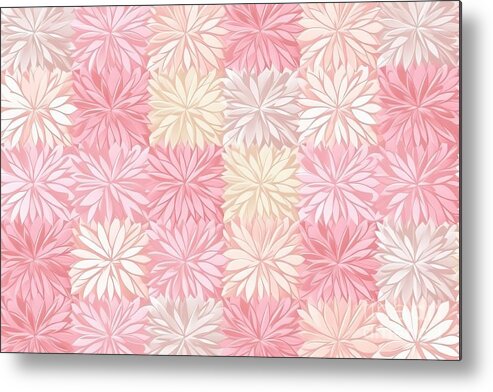This digital painting features a meticulously arranged floral pattern, framed by a thin black border approximately one pixel wide. The artwork displays a grid of 30 chrysanthemums, precisely organized into five rows and six columns. Each flower, while identical in shape, varies in color, presenting a spectrum from almost white and ivory to light pink and dark pink hues. The colors are distributed randomly, creating a captivating and visually appealing pattern. The overall composition, with its soft transitions between shades of pink, white, and beige, makes for an elegant piece of wall art that adds a touch of grace and tranquility to any space.